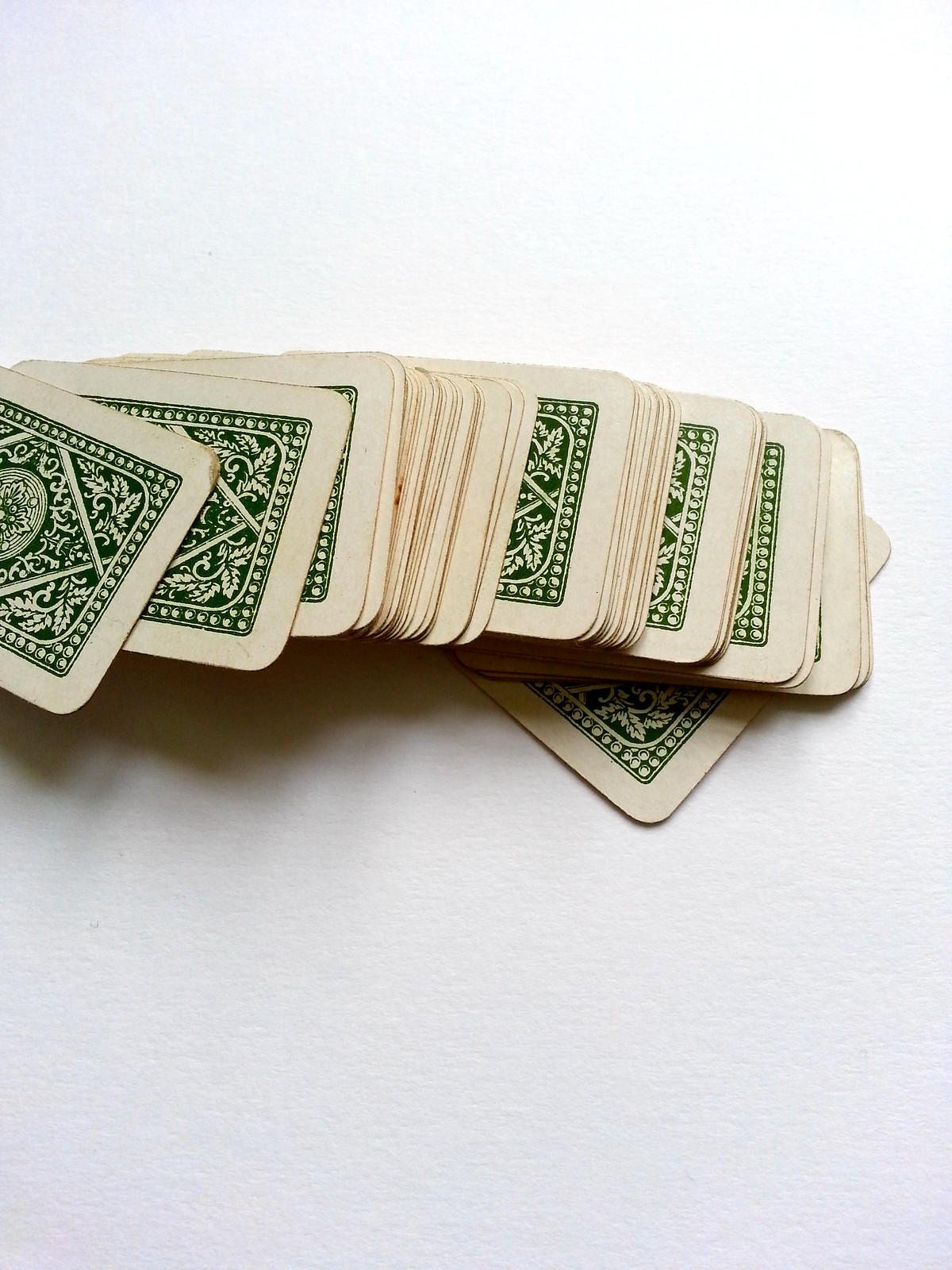This photograph captures a set of playing cards arranged against a pristine white background. The cards are depicted from the back, meticulously fanned out in a staggered fashion towards one side. The predominant color of the cards is white, but their backs reveal an elegant green design replete with intricate details. 

The green section showcases a blend of white and green elements resembling leaves and lines, culminating in a circular motif at the center. Within this circle, delicate lines converge to surround what appears to be either a floral pattern or foliage, accented by tiny circles along the lines. The border surrounding the green area is adorned with miniature white dots, reminiscent of BB pellets, subtly tinged with green shading to enhance their appearance.

Despite the overall pristine arrangement, the cards exhibit signs of wear. The top card on the left side, for instance, has a discolored, brownish corner. Additionally, midway through the deck, some cards display brown edges, further emphasizing their used and aged condition.